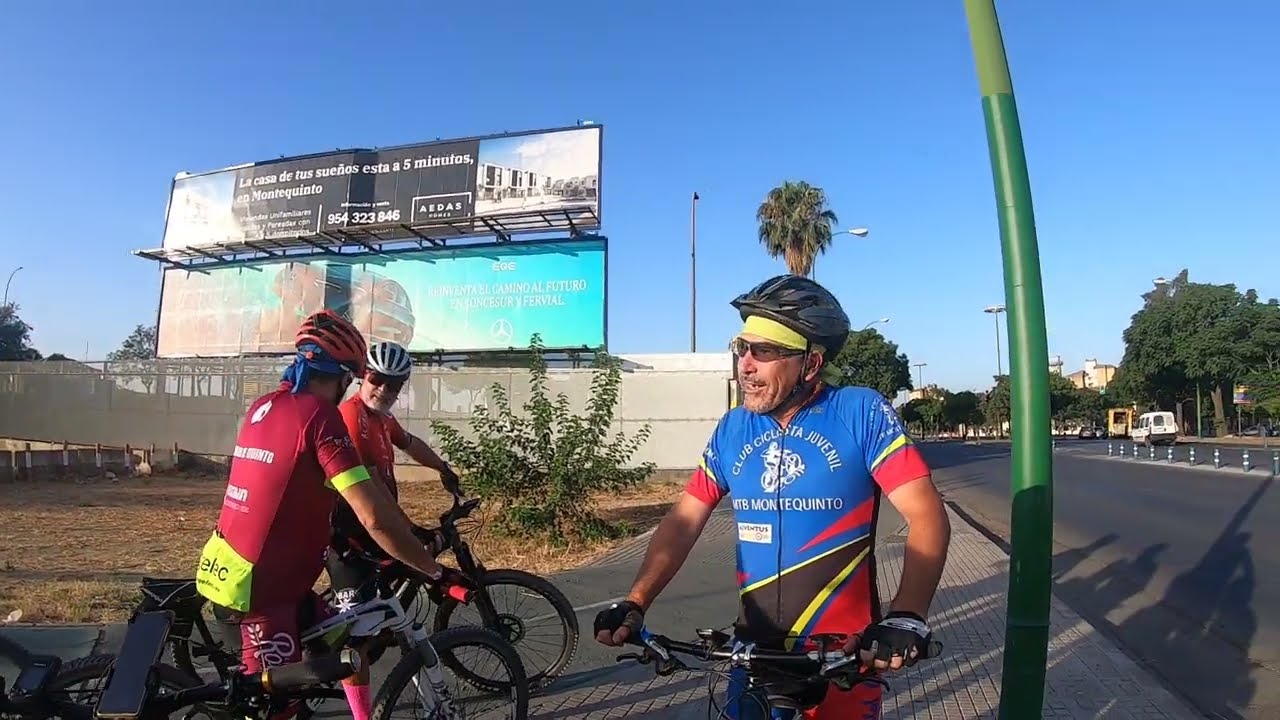The image, taken on a sunny day, depicts three cyclists dressed in biking outfits, likely participating in a biking event or convention. They are positioned near a street corner, and the sun casts clear shadows indicating bright conditions. Two cyclists in red attire are on the left side of the image, engaged in conversation and facing towards the right. A third cyclist, wearing a blue outfit with various colors, is positioned slightly apart, looking towards the left. They are all on black bicycles.

A green electrical pole and a streetlight pole are visible near them, indicating their position on a sidewalk adjacent to a roadway. In the background, there are two billboards, one of which is partly legible with Spanish text. A scrubby bush is close to the two cyclists on the left, while some palm trees and parked cars line the road, indicating a tropical or beachside location. To the right, there's a white fence and additional trees, enhancing the outdoor setting.